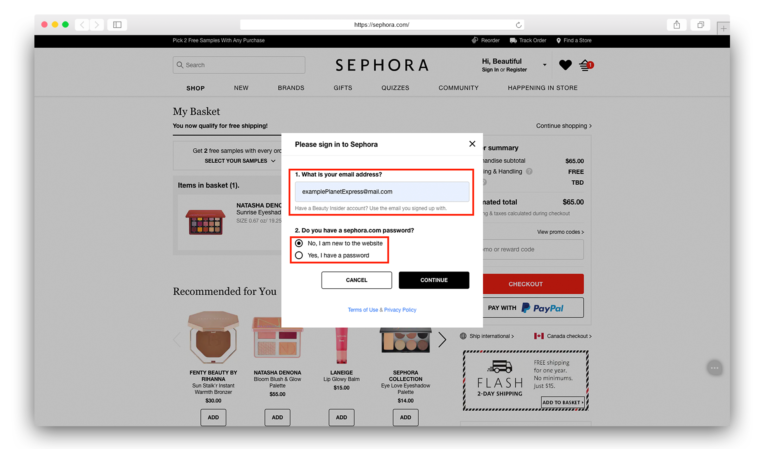The image is a computer screenshot with a gray background and a header bar at the top. Centrally positioned on the screen is a white rectangle functioning as a search bar. Above the search bar, centered and displayed in bold black letters, are three words. Below this, a thick black horizontal rectangle spans the width of the screen. Further down, centered and in bolded black all caps with spaces between each letter, it reads "SEPHORA."

In the middle of the screenshot is a prominent white square. In the upper left-hand corner of the square, it says "Please sign in to Sephora" in bold black text. Beneath this statement are a couple of input boxes and buttons positioned at the bottom of the square. Overlaying this, in the background, is the main Sephora website interface displaying various beauty products.

On the overlayed Sephora screen, the top left corner displays the words "My Basket" in gray. To the right are listed prices, and below are recommended products. Notably visible are images of eyeshadow and lipstick. At the bottom of the screen, there is another black rectangle, outlined with slanted black lines. Inside this rectangle, on the left side, there is an image of a truck with the word "FLASH" underneath, written in all caps gray with spaces between each letter.